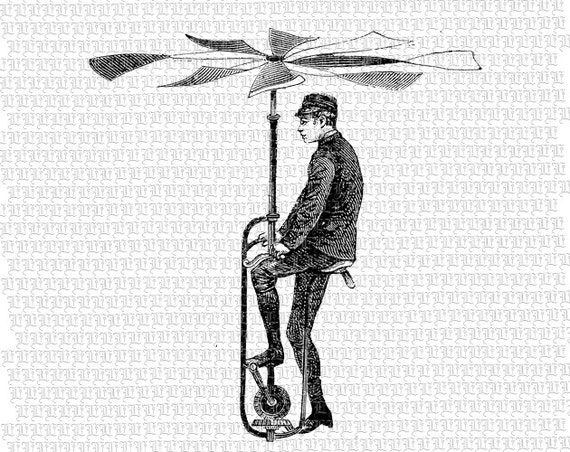This detailed illustration in black and white showcases a vintage, early 20th-century flying machine concept. The central figure, a gentleman adorned in a black suit, black shoes, and a bellhop-style cap, is depicted from a side angle as he pedals a unicycle-like apparatus. One foot rests on the pedal while the other appears to be on the ground. The machine features a single wheel and a complex structure of tubes and bars connecting to a central pipe overhead. Topping this pipe are eight fan-like blades, suggesting the intent to achieve flight through pedal power. The entire scene is rendered in ink or pencil with a pale gray and white patterned background that includes various geometric shapes or possibly ornate letters, giving a textured, animated feel to the backdrop.